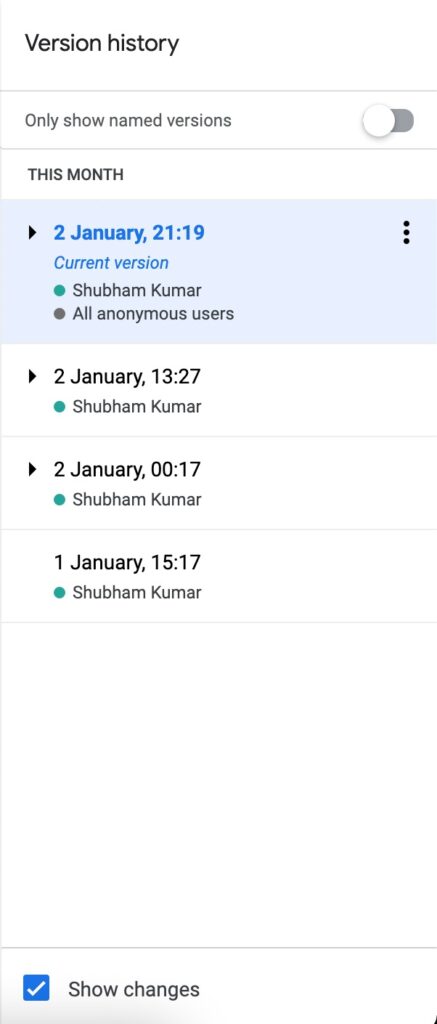The image portrays a web page optimized for viewing on mobile devices, such as phones or tablets, displaying a version history interface. The page features a minimalist design with a white background and predominantly black text. 

At the top left corner, the text "Version History" is prominently displayed. Directly below this header is an option labeled "Only show named versions," next to which is a toggle slider that is currently set to "off." This section is visually separated by two horizontal lines, one above and one below the "Only show named versions" text.

Below this, the phrase "This month" serves as a subheading. Beneath this subheading is a light blue shaded rectangle with a small blue arrow pointing to the left. The text inside the rectangle reads "2 January 21:19," followed by "Current Version" in black text, attributed to "Shuman Kumar" with an additional note indicating contributions from "all anonymous users." To the right of this line, three vertical dots indicate additional options.

Further down the page, there is a chronological list of version logs against the same white background. Each entry shows a timestamp and the name "Shuman Kumar":
- "2 January 13:27"
- "2 January 00:17"
- "1 January 15:17"

Each of these entries is separated by horizontal grey lines for clear distinction.

Towards the bottom of the image, there is a noticeable white space followed by another horizontal grey line. Below this line is a blue checkbox labeled "Show changes," which is currently checked. The checkbox also casts a subtle shadow underneath.

There are no additional icons or images on the page; it solely displays the version history details in a clean and organized manner.